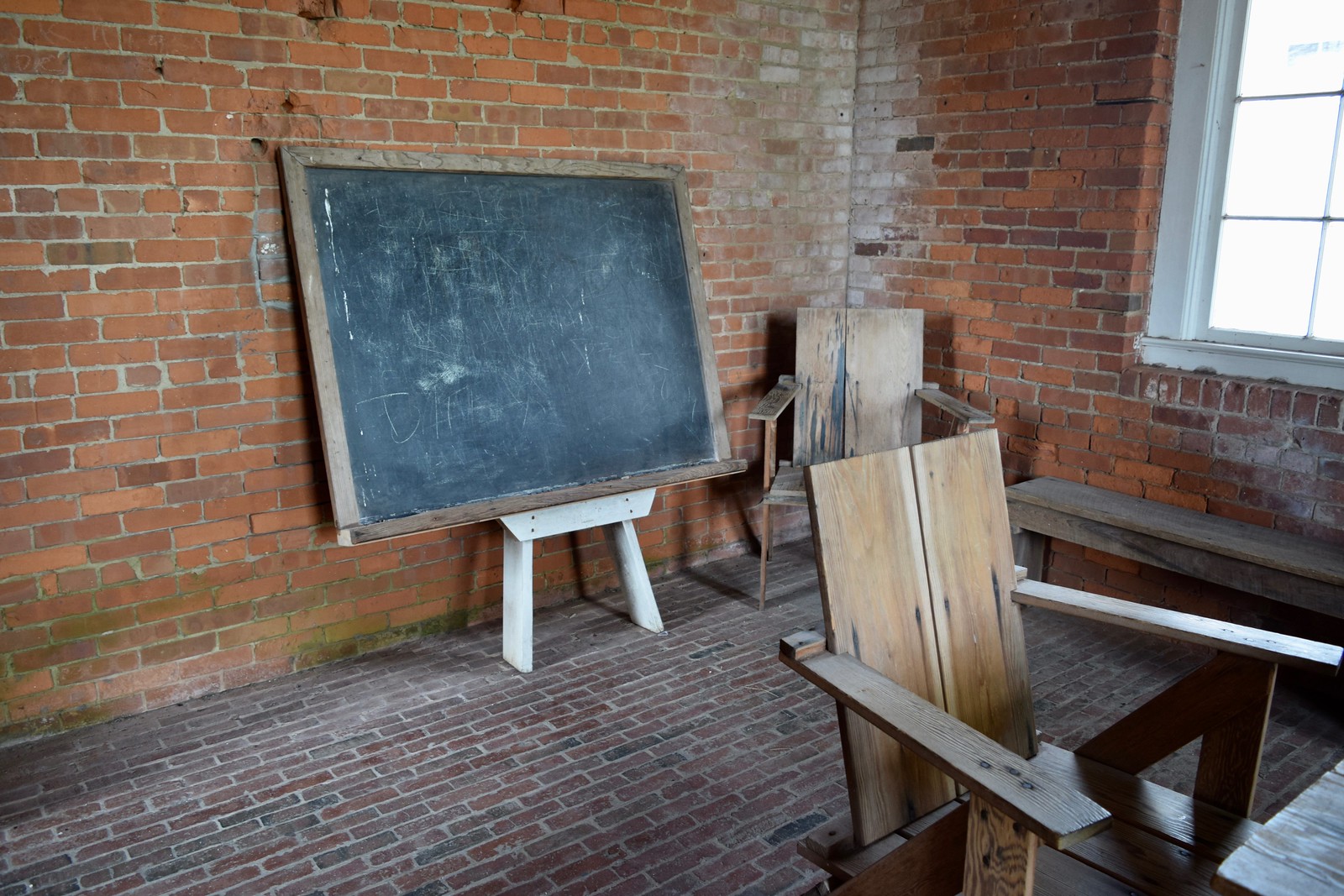The image captures an interior storage-like room with distinct elements and rich details. Central to the photo is a black chalkboard with a brown trim, perched on a white stool and leaning against a red brick wall. The floor is constructed from similarly hued bricks, adding to the rustic feel. In the corner, there's a wooden chair facing the right, accompanied by a second wooden chair positioned towards the center of the photo. To the right, near a white-trimmed window with clear glass panels, lies a wooden bench. The window suggests it's daytime as sunlight filters through. Additionally, some portions of the red brick wall are stained with white. A picnic table appears to be laying on its side in the foreground, contributing to the room's storage atmosphere.